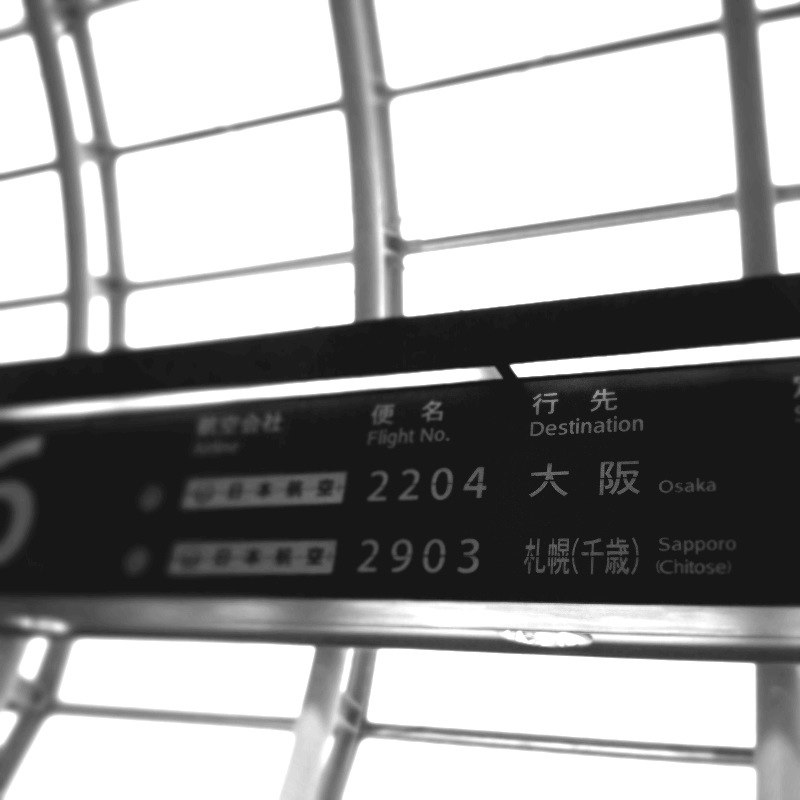The black and white close-up image captures a striking scene at a Japanese train station, showcasing a prominently centered black sign with Japanese and English text. The environment is minimalist, devoid of people, accentuating the gleaming metal framework that supports the sign. This intricate metal grid, with both vertical and horizontal elements that curve slightly like blinds, adds a sophisticated touch to the composition. Central to the sign are striking Japanese characters indicating "BINNA" and "YUKI", flanked by the English words "Flight Number" and "Destination". Two specific flight numbers, 2204 to Osaka and 2903 to Sapporo (Chitose), are clearly displayed. On the left side of the image, a partially obscured column adds a touch of mystery, blending into the blurred background.